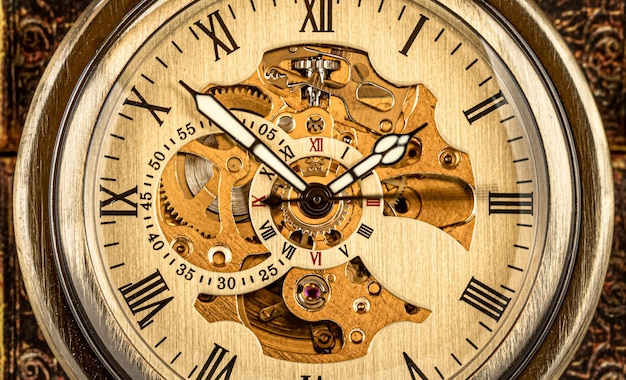This image is a detailed close-up photograph of a clock with a predominantly light wood aesthetic. The clock face and frame are made of a light-colored wood, with Roman numerals marking the hours from 1 to 12. The face also features black lines indicating the minutes and seconds. The clock dials are distinct with a white surface outlined in black metal. At the center of the clock, there's a ring of the same light wood as the face, which also includes the Roman numerals. An inner disc displays additional numbers, and the remainder of the clock is transparent, showcasing its intricate gold-colored springs and gears. The ornate background of the clock appears to be made of gold or brass, adding to its decorative appeal. The clock appears to be cut off at the top and bottom in the photograph. The hands of the clock point to approximately 1:52 p.m., adding a dynamic element to the captured image.